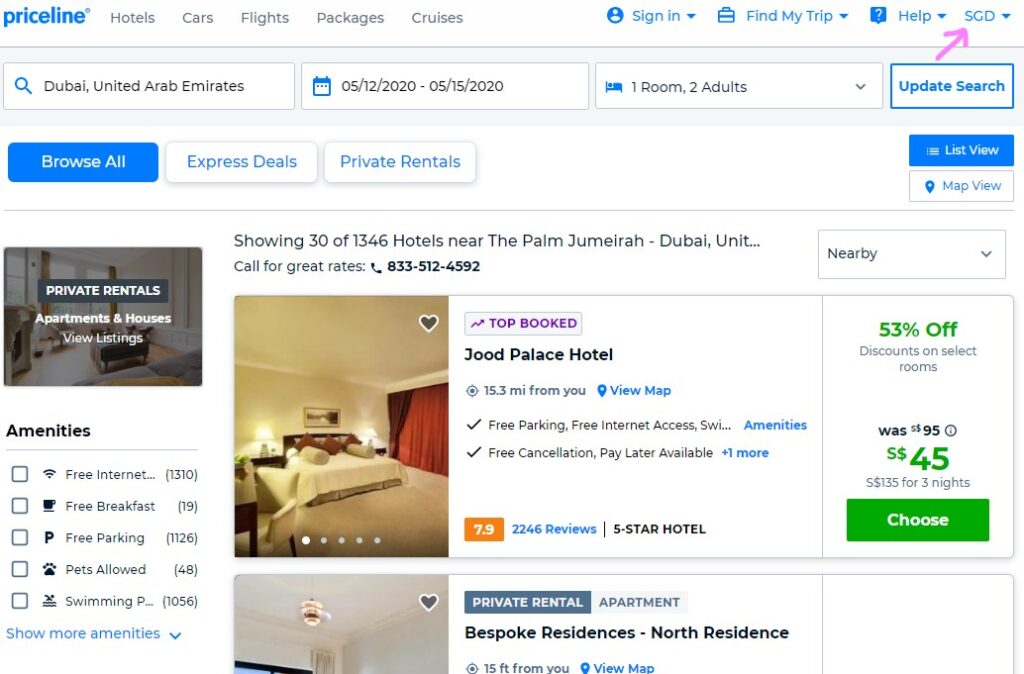The image displays a Priceline webpage, prominently featuring the Priceline logo with a registered trademark symbol in blue. The top navigation bar, from left to right, includes options for hotels, cars, flights, packages, cruises, sign in, find my trip, help, and SCD. Beneath the navigation bar, there's a section indicating a search query for "Dubai, United Arab Emirates," with travel dates from May 12, 2022, to May 15, 2022. The search is for one room accommodating two adults. To the far right, there's an "Update Search" button.

Directly below, a bright blue button labeled "Browse All" is positioned alongside white buttons for "Express Deals" and "Private Rentals." On the right side, options for "List View" and "Map View" are available. Further down, a room advertisement highlights "Private Rentals, Apartments and Houses," with a "View Listings" link.

In the center of the page, a section announces "Showing 1346 hotels near Palm Jumeirah, Dubai." Alongside this, there is a promotion stating "Call for Great Rates" with a phone icon and the number 833-512-4592.

A specific hotel listing for the "Jude Palace Hotel" is featured, indicating it is 15.3 miles from the searcher’s location and available to view on the map. The hotel offers amenities like free parking, free internet access, free cancellation, and the option to pay later. It has garnered 2246 reviews, achieving a 5-star rating with an average score of 7.9. To the right of this listing, a highlighted discount shows a 53% reduction in price, originally $95, now $45 per night, totaling $135 for three nights. A green button invites users to "Choose."